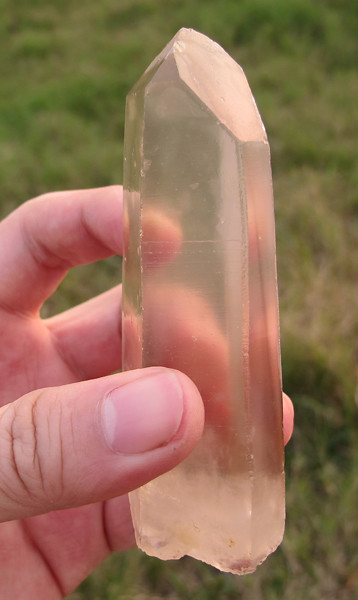The image is a rectangular outdoor photograph taken in natural light, likely around sunset, as suggested by the warm glow. The background is predominantly green, indicative of a grassy field with some weeds, and a patch of brown dirt is also visible on the right side. The focal point is a close-up view of a man's strong hand with short, jagged fingernails holding a large crystal. The crystal, about the height of a cigarette pack but narrower, has a rose-gold hue and is elongated with a pointed top resembling a dagger. It features a smooth, polished surface at the top, cut at an angle, while the bottom exhibits a jagged texture.